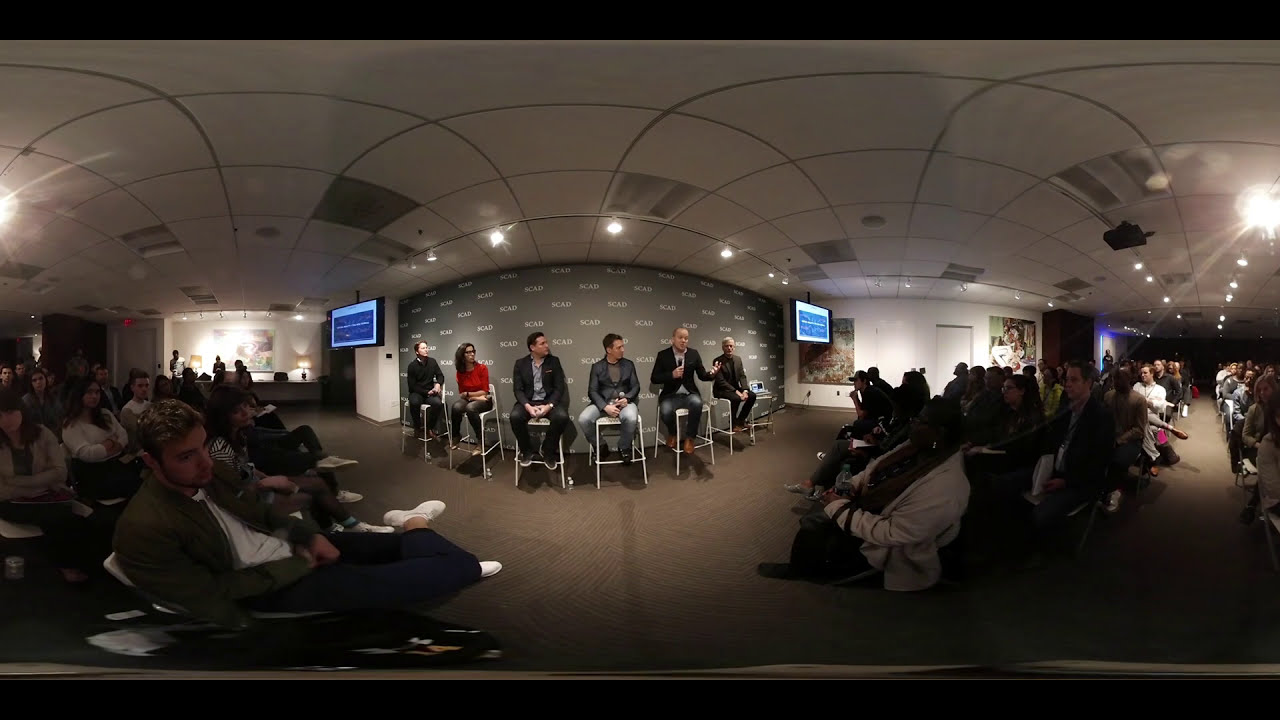This image depicts a conference or press event taking place in a large room. The picture is a wide horizontal rectangular shot, framed by thin black stripes on the top and bottom edges. The focal point is a group of six individuals, five men and one woman, seated on stools lined up against a gray wall. These people are dressed in business attire—suit jackets and pants. The second individual from the right, a man wearing a black jacket, white shirt, gray jeans, and brown shoes, is holding a microphone and appears to be addressing the audience with expressive hand gestures. The remaining members of the group are attentively watching him.

Behind the speakers, the gray wall features the white text "SCAD." Mounted on either side of this group are TV screens displaying unreadable white text against blue backgrounds. The ceiling comprises white and gray square panels with built-in lighting. The room is expansive, hosting an audience seated in multiple rows of chairs. Although the attendees are not well-lit and individual details are hard to discern, some audience members are visible: one person in the front left wears a green coat, white undershirt, blue pants, and white shoes, while a woman across from him wears a white coat, brown undershirt, and black pants.

Additional lighting fixtures and ceiling panels are visible, and there are posters on the walls. The overall setting is an indoor venue arranged for a formal event, emphasizing the speakers and the attentive audience.